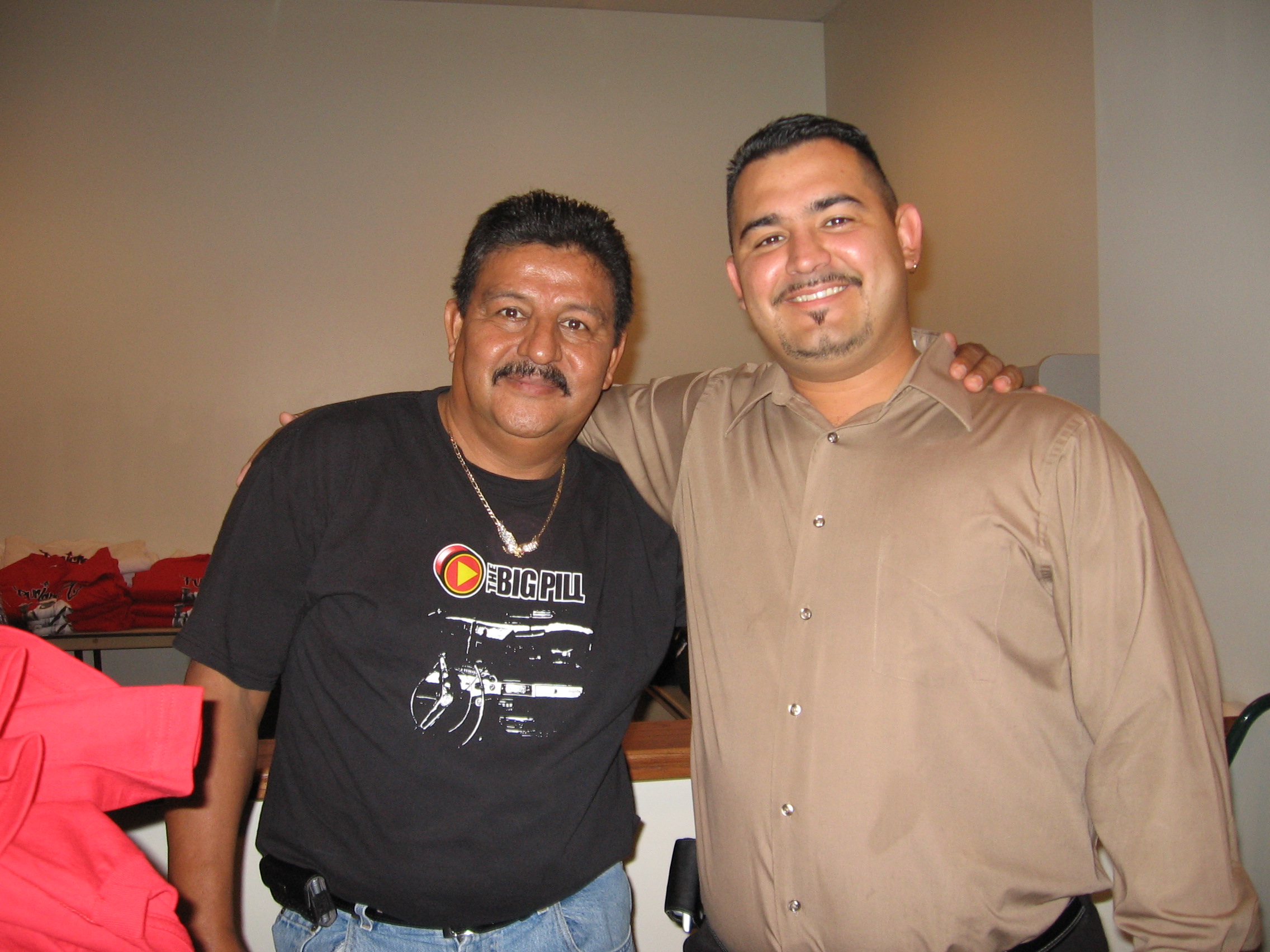In the image, two Hispanic men with brown skin and short black hair are standing close to each other, arms around one another in a friendly embrace. Both men are smiling broadly, and they each have mustaches. 

The man on the right has shorter hair and is adorned with a small earring in one ear. He sports a meticulously trimmed short goatee and wears a buttoned-up, long-sleeved brown shirt with a collar. On his belt, he has either a cell phone case holder or a beeper holder.

The man on the left is dressed in a black t-shirt displaying the words "The Big Pill" alongside a distinctive play button logo featuring a yellow triangle within a 3D red circle and a small white design. Around his neck is a chain, and on his belt, he also has a cell phone case holder or beeper. 

Behind them, the setting features brown-colored walls and a table neatly arranged with folded clothing, including prominently visible red shirts.